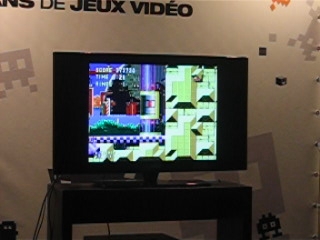The image captures a vibrant scene from a video gamer's paradise, likely set at a gaming expo or a themed event dedicated to the love of video games. Dominating the scene is a flat-screen television, prominently displaying a classic platform video game complete with nostalgic, pixelated graphics that harken back to the golden age of console gaming. The game itself features a lively outdoor setting with various platforms, obstacles, and colorful characters typical of early video game design.

Above the TV, a partially visible banner reads "Jeux Vidéo," the French term for "Video Games," indicating that this exhibit is part of a French-speaking event or location celebrating the culture and history of video gaming. The television sits neatly on a simple, unassuming black stand, allowing the viewer’s attention to be focused entirely on the vibrant screen. Surrounding the setup, the background is tastefully adorned with pixel-style decorations, enhancing the retro gaming atmosphere and immersing attendees in the nostalgic world of classic video games.